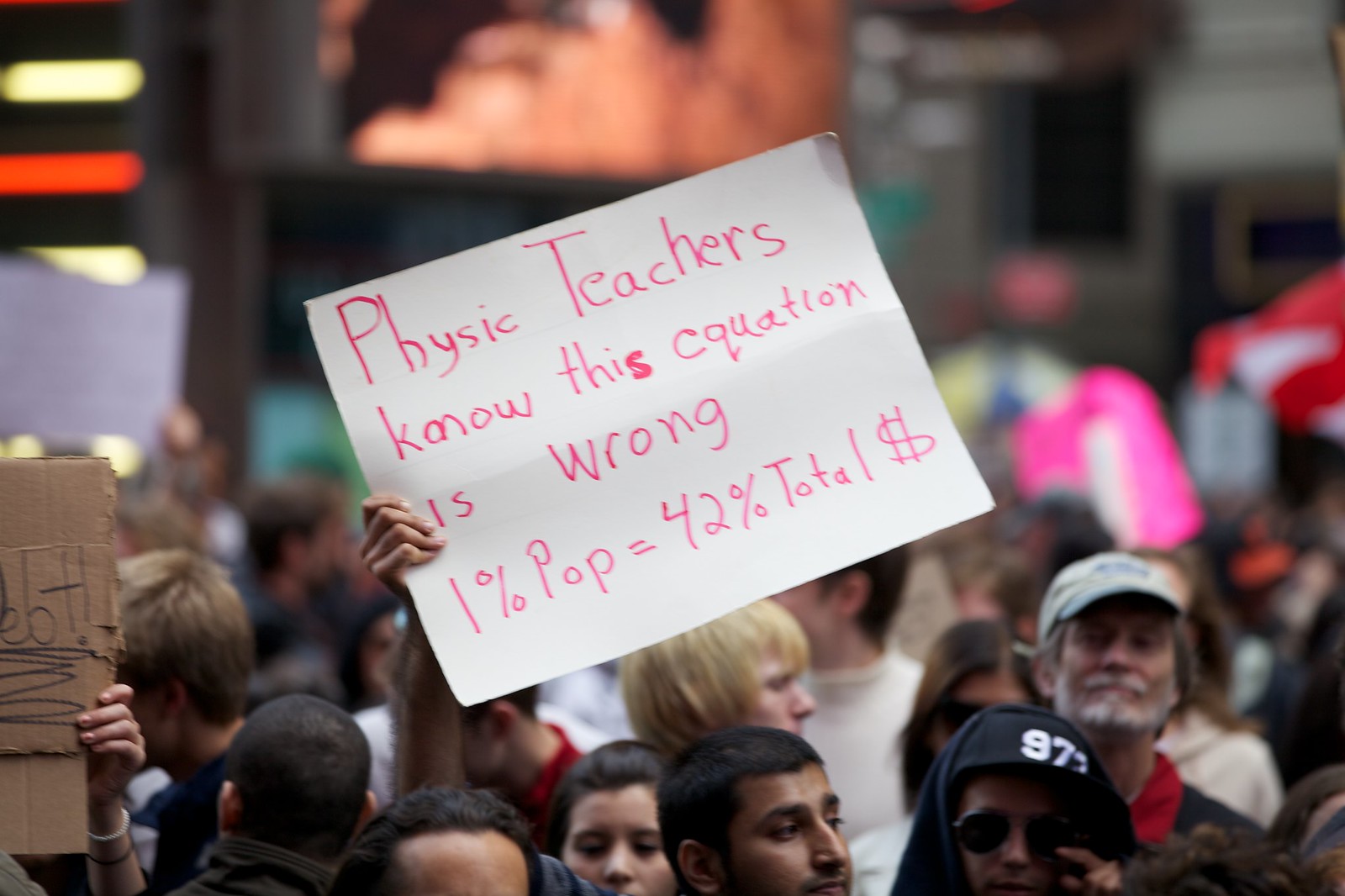The image captures a vibrant outdoor economic inequality protest rally, characterized by its photographic style and detailed composition. Dominating the foreground is a sign held by an individual, containing the provocative message written in pink: "Physics teachers know this equation is wrong, 1% of the population equals 42% of total dollars." This sign is tilted upwards diagonally, and it is held by a young man, possibly of Indian descent, standing to the left of the center. Surrounding him, the diverse crowd includes a young blonde man, whose face is partially visible above a young Hispanic man, a white man wearing a black baseball cap with the number 97, and a white woman with black hair.

In the far-left corner, another protester holds a cardboard sign that reads "EBT!" with only their white hand visible. The background includes several people who become blurrier as they recede, with some holding red, white, blue, yellow, and possibly pink umbrellas. The scene is set against a backdrop of blurred buildings adorned with indistinct billboards, adding to the bustling atmosphere of the protest. Additionally, on the right side of the image stands an older man with a gray beard, wearing a light blue hat and a red collared shirt, observing the rally.